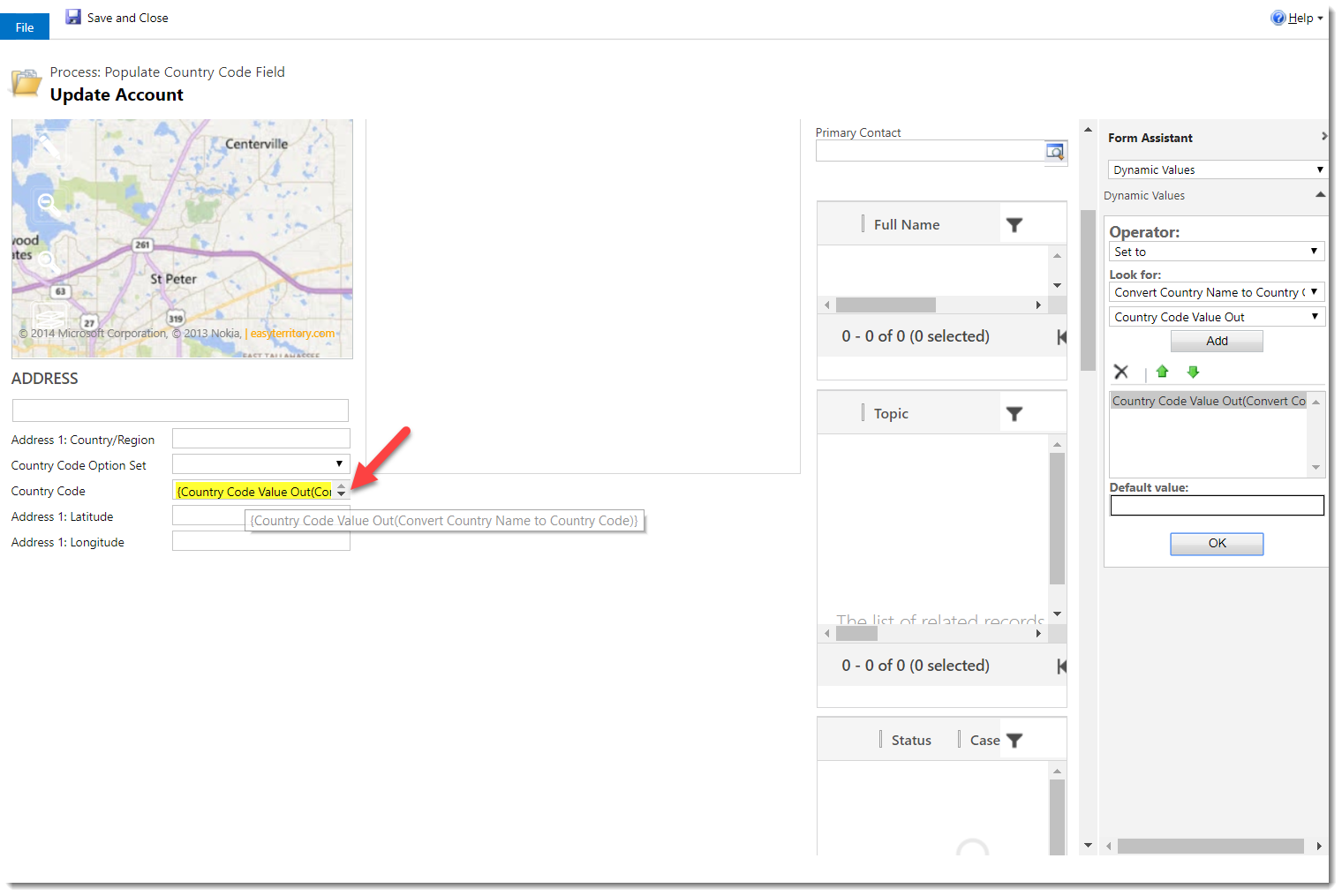This image features a detailed interface layout, resembling a data entry map with various options for input and storage. In the upper left corner, there is a blue rectangular button labeled "File," followed by "Save" and "Close," accompanied by a blue save icon. On the upper right, there's a "Help" dropdown menu.

The central body of the interface contains instructions for processes like populating a country code field and updating an account. A small 2014 Microsoft Corporation map displays cities such as Centerville and St. Peter, with identifiable highways 261, 63, 27, and 319 marked by blue lines.

Here, users can input addresses with designated text fields for "Address One" and "Country/Region," as well as dropdown options for "Country Code." Further fields include "Address One Latitude" and "Address One Longitude." 

On the right side, fields are available for entering "Primary Contact," "Full Name," "Topic," and "Status," all presented as text boxes. Additional options include a dynamic selection for "Inform Assistant," dropdowns for "Operator" setup, and selections to "Look for" specific criteria. Users can also use dropdowns to convert country names to corresponding country codes or values.

Overall, this interface appears to be designed for comprehensive data input and geographical information management.